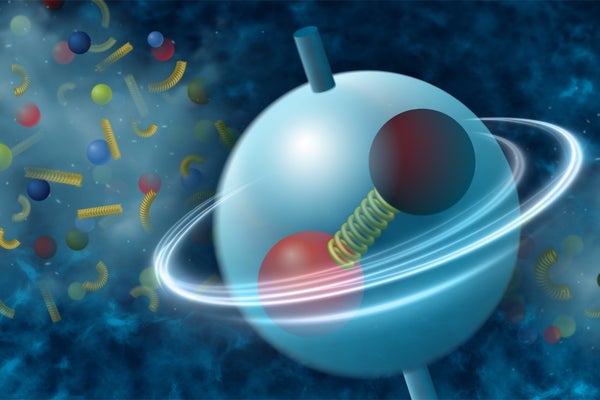The image appears to be an AI-generated illustration likely depicting a microscopic or scientific scene. The background features a light blue area on the left side with light beams, transitioning into darker blue shades towards the top, bottom, and right. Scattered throughout the image are various colorful objects, predominantly spheres in red, blue, lighter blues, greens, and near-yellow hues resembling macaroni shapes.

Dominating the center of the composition is a light blue sphere resembling a planet, complete with white rings encircling it. A vertical pole runs through this central sphere, which further contains an internal structure resembling a dumbbell with a yellow spring as its handle. To the right side of this central sphere lies a black ball, while a red ball is located to its left. The smooth details and diverse color palette suggest the image's purpose may be educational, possibly for a textbook or other scientific illustration.